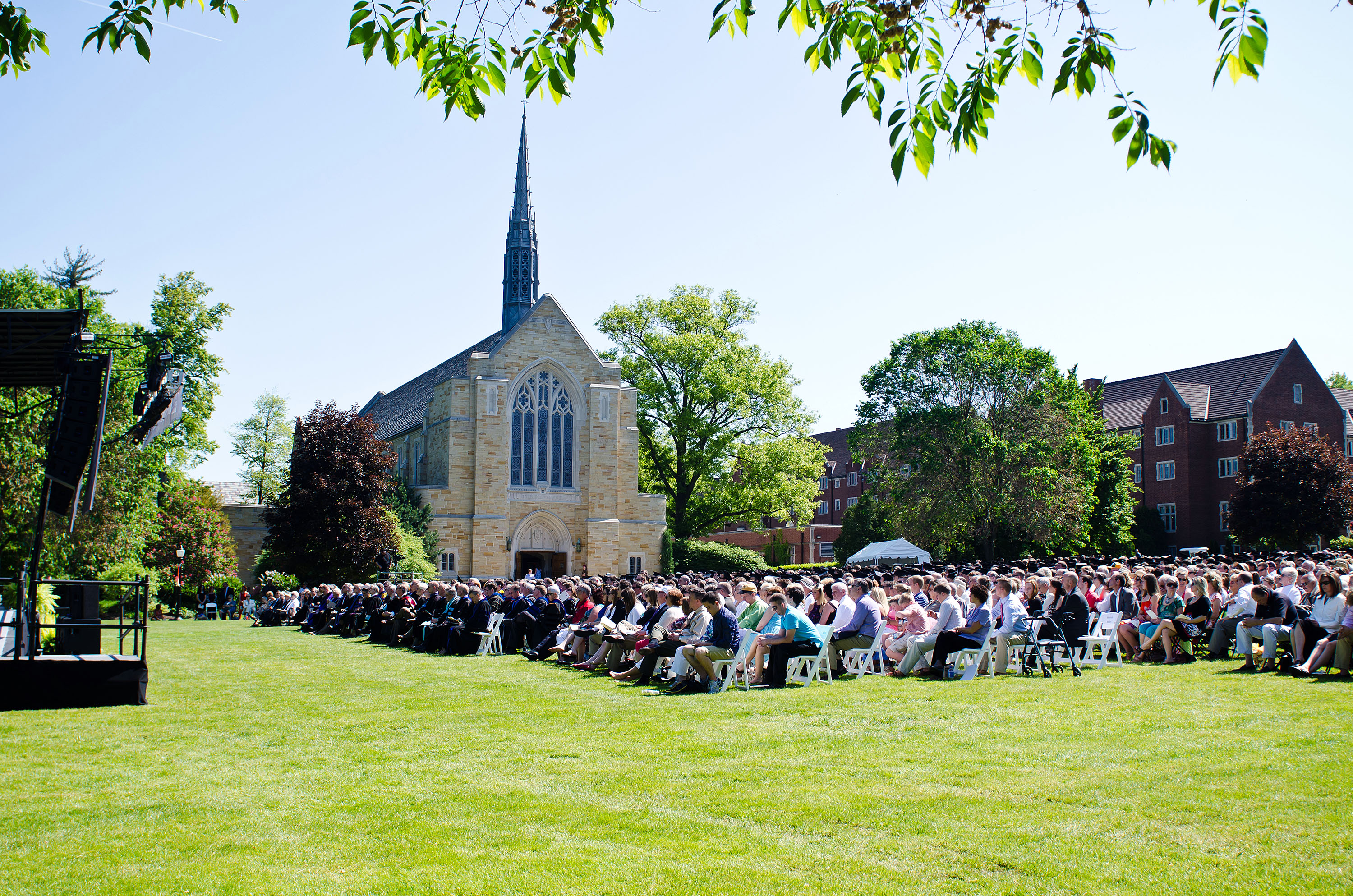The image captures a vibrant outdoor setting on a bright, blue-skied day, although the sun itself isn't visible. Dominating the background towards the center-left is a grand church or cathedral, flanked on the right by a long, dark red brick building. The foreground is filled with a large grassy area where numerous people are seated on chairs, dressed in varied attire. Among them, near the church, a group donning graduation gowns stands out, suggestive of a commencement ceremony, while to the right, spectators in more casual clothing are visible. A black stage is noticeable to the left side of the image, with everyone appearing to be facing its direction. Leafy trees dot the scenery and branches with light green to brown leaves drape across the top of the image, adding a natural canopy.